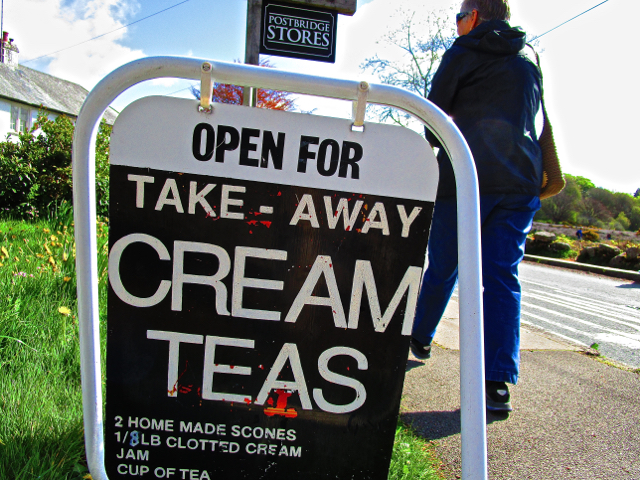In the image, an outdoor scene features a circular sign prominently mounted on a white-painted pipe set in a grassy area. The sign, which is framed with a white border, bears text in black and white. At the top, it reads "Open for Takeaway Cream Teas" in black and white lettering. Below, in smaller text, it offers details about the treat: "Two homemade scones, 1/8 lb clotted cream, jam, and a cup of tea." The sign appears slightly weathered and is attached to two metal bars.

To the left of the sign, there is additional signage reading "Postbridge Stores." A narrow path or pavement runs alongside the grassy area on the right, where a woman dressed in a coat and blue trousers, with a handbag on her right arm, walks by. Further surroundings include a white house with a grey roof in the top right corner, under a clear blue sky scattered with a few clouds. Green vegetation is visible on the opposite side of a grey road which has some white markings. The setting hints at a residential neighborhood in England, captured during the daytime, possibly mid to late evening based on the shadow angles.